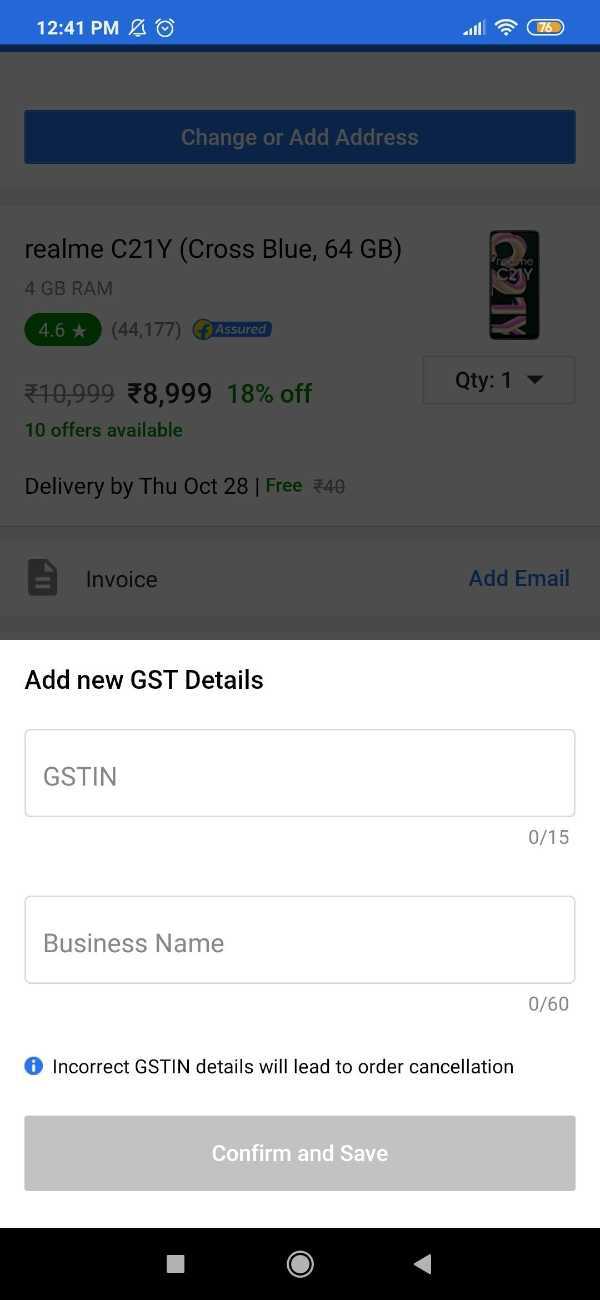A screenshot from a phone at 12:41 PM showcases various elements of an online shopping interface. The top section displays a blue banner with the time on the left, notifications turned off, and an alarm icon. On the right, there are four Wi-Fi bars indicating full connectivity and a yellow battery icon showing 76% charge. The main window has a translucent gray overlay, giving it a dark appearance. 

At the top of the main content area, a dark blue horizontal banner states "Change or add address" in white text. Below this, in black text, is the product description: "Realme C21Y Cross Blue, 64GB, 4GB RAM" accompanied by a rating of 4.6 stars based on 44,177 reviews, and a tag indicating it is "Assured." A thumbnail image of the phone is displayed to the right, with the quantity set to one.

Beneath the product details, the price is shown as $8,999 in black, with a green text indicating "18% off" and "10 offers available." The delivery information states, "Delivery by Thursday, October 28th is free." The bottom left of this section features an "Invoice" link, while the bottom right shows an "Add Email" option.

Further down, the interface prompts the user to "Add new GST details." There are text boxes for GSTIN and business name, followed by a warning note that incorrect GSTIN details will lead to order cancellation. A gray bar at the bottom highlights a white "Confirm and Save" button. The very bottom of the screen includes the close, minimize, and back buttons.